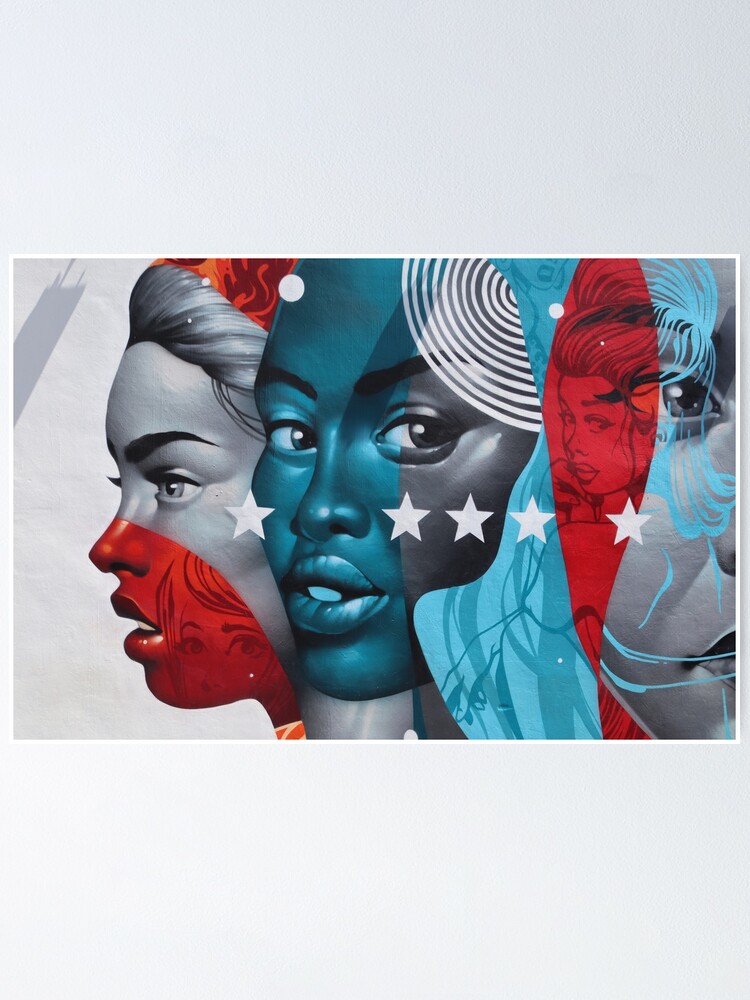This striking poster features three female faces arranged in a futuristic, artistically stylized manner. The image is predominantly in shades of gray, black, and white, with vibrant splashes of red and blue. On the left, one woman looks to her left, her face gray with the lower half colored bright red, which also contains a tattoo-like image. In the center, a darker-gray-skinned woman gazes slightly towards the front; her face is partially covered in blue. To the right, another woman looks to her right, showing only half her face—partially obscured by a red section featuring another tattoo-like depiction. The background is gray, and five white stars stretch across the middle of the composition, adding a striking visual element. The entire piece has a computer-generated feel, blending artistic flair with a touch of modern aesthetics.